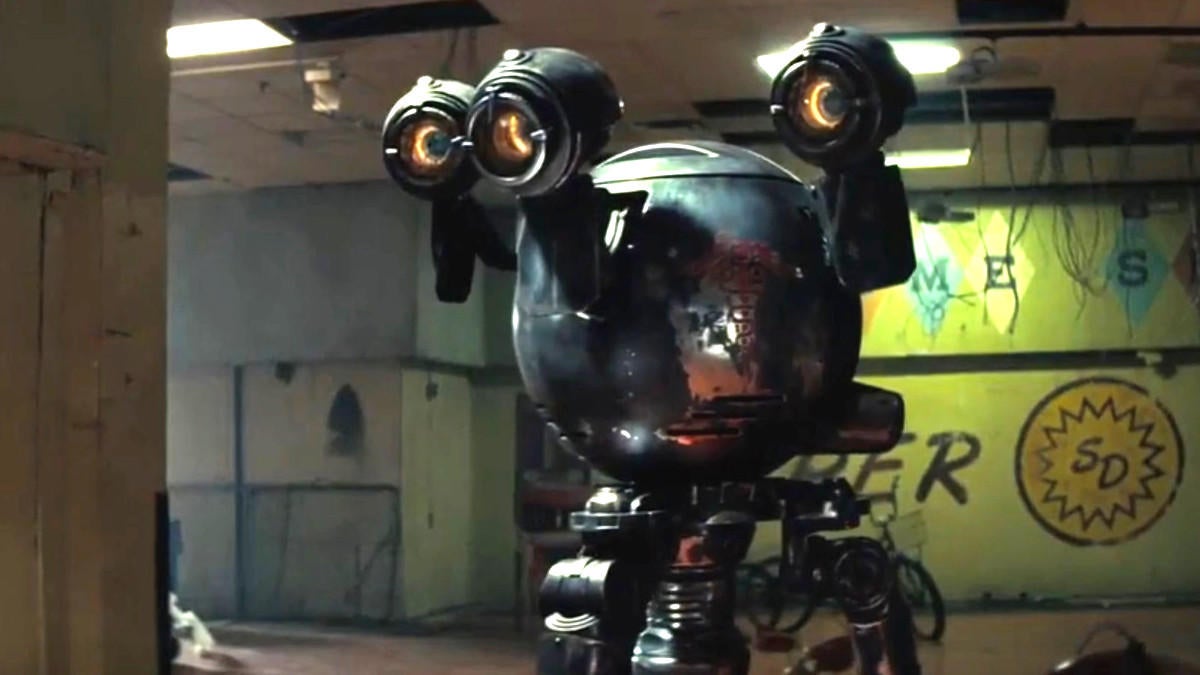In this detailed photo from the Fallout TV show, we see Mr. Handy, a recognizable robot from the Fallout series. The robot has a large, dark metallic orb as a body with three protruding, camera-like eyes. The eyes are yellowish in color with black irises. Mr. Handy's exterior shows signs of wear, with red graffiti on one side and patches of exposed metal. The robot's three legs extend from a central joint, giving it an almost octopus-like appearance, with two legs positioned in the front and one in the back.

The setting appears to be a dilapidated building, characterized by its worn and damaged state. The background features a yellow wall adorned with various details. The word "P-E-R" is visible, suggesting it could be part of the word "super." A black circle with a sunburst symbol, complete with numerous spikes and the letters "S-D" in the center, is also noticeable. The upper portion of the wall displays a series of diamonds: a blue diamond with an "M," a yellow diamond with an "E," a space, and another blue diamond with an "S." Additionally, numerous wires dangle from the ceiling, further emphasizing the building's ruined condition.